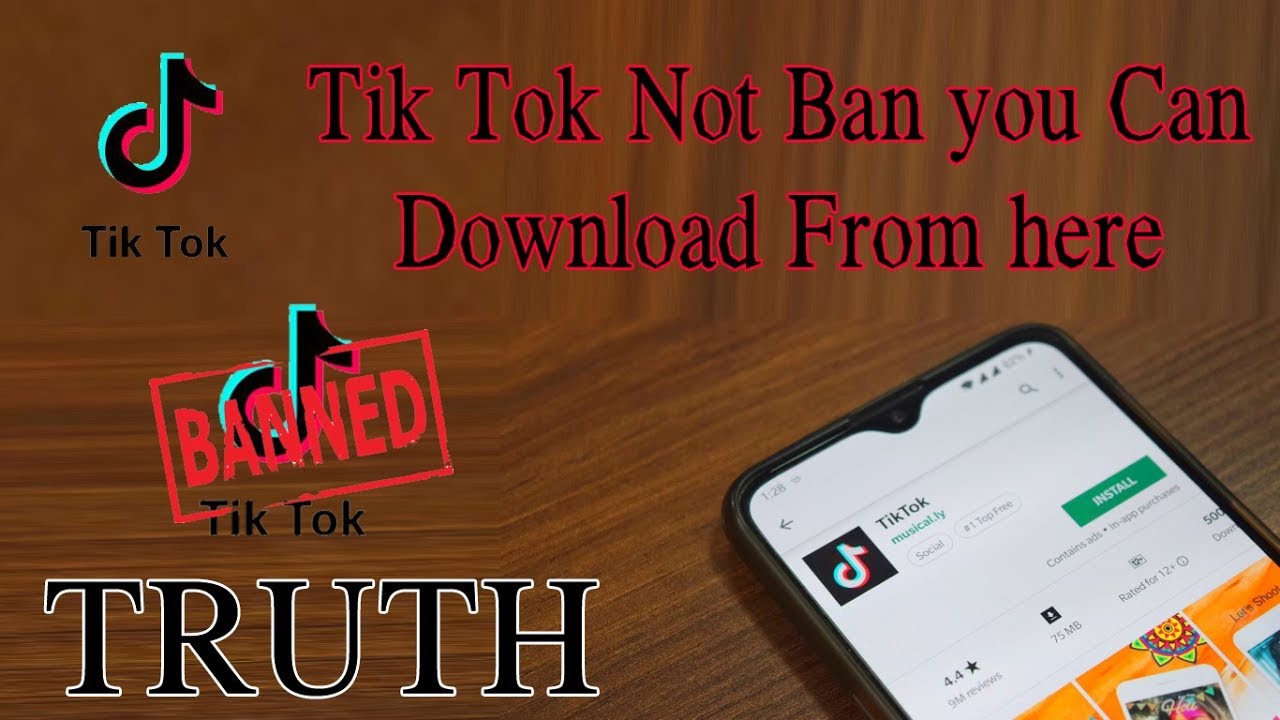The image features a brown textured background with various elements and texts. At the top, the text "TikTok Not Banned" is prominently displayed in black with a red outline. To the left of this text, there is the iconic TikTok logo, which consists of a black music note with blue and red accents. Below the top text, the word "TikTok" appears again in black.

Towards the bottom left corner, another TikTok logo appears with a red stamp over it that says "Banned." Directly beneath this logo, the word "Truth" is written in bold black letters with a white outline.

In the bottom right corner, there's an image of a black smartphone displaying the Google Play Store app. The app visible on the screen is TikTok, represented by its logo—a music note with a black background. To the right of the logo, the text "TikTok" is displayed, followed by "musical.ly" and "Social, Number 1 Top Free." A green button labeled "Installed" is located beneath, indicating that the app is already downloaded. The TikTok app is shown with a 4.4-star rating, 9 million reviews, 75MB size, and a rating appropriate for ages 12 and up.